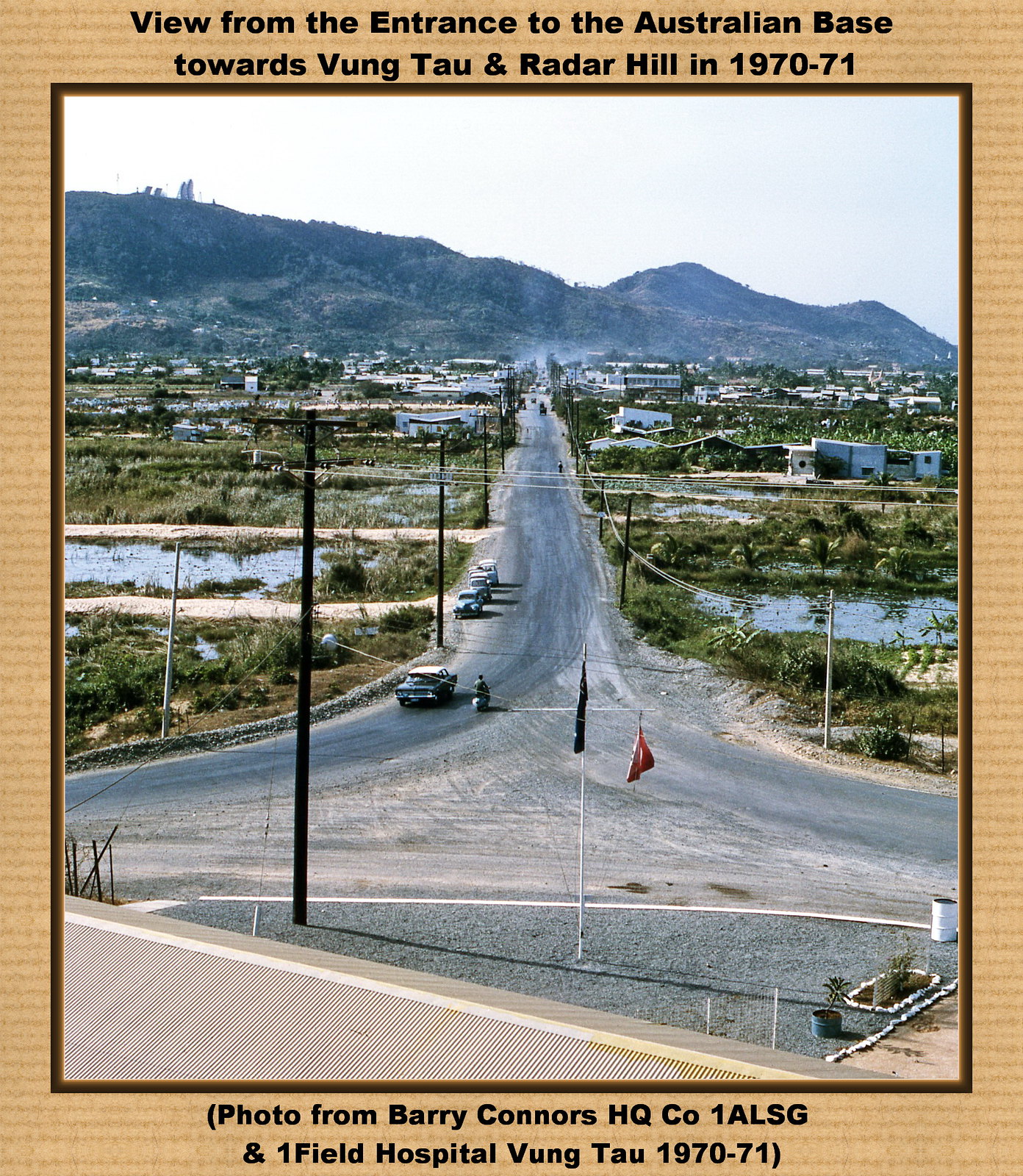The photograph is mounted on a cardboard-like border with a beige hue. The top of the border features bold black text that reads: "View from the entrance to the Australian base towards Vung Tau and Radar Hill in 1970-71." Below the photograph, there is further black text stating, "Photo from Barry Connors HQ CO 1ALSG and Onefield Hospital Vung Tau 1970-71."

The image itself captures a panoramic outdoor scene from the entrance of the Australian base. In the foreground, two flagpoles stand prominently, one bearing a blue flag and the other a red flag. A road cuts through the center of the village, with a few cars and a motorcycle visible on it. The road eventually parts, heading in eastern and western directions. On either side of the road, rows of modest houses are interspersed with patches of green shrubbery and small drainage ponds or ditches filled with water. Utility poles line the road, leading the eye towards the middle ground and further emphasizing the depth of the scene.

In the background, rolling hills and mountains rise under a light, hazy sky, creating a tranquil yet structured landscape. The overall mood of the photograph is nostalgic, capturing a moment in time during the years 1970-71 with detailed precision.